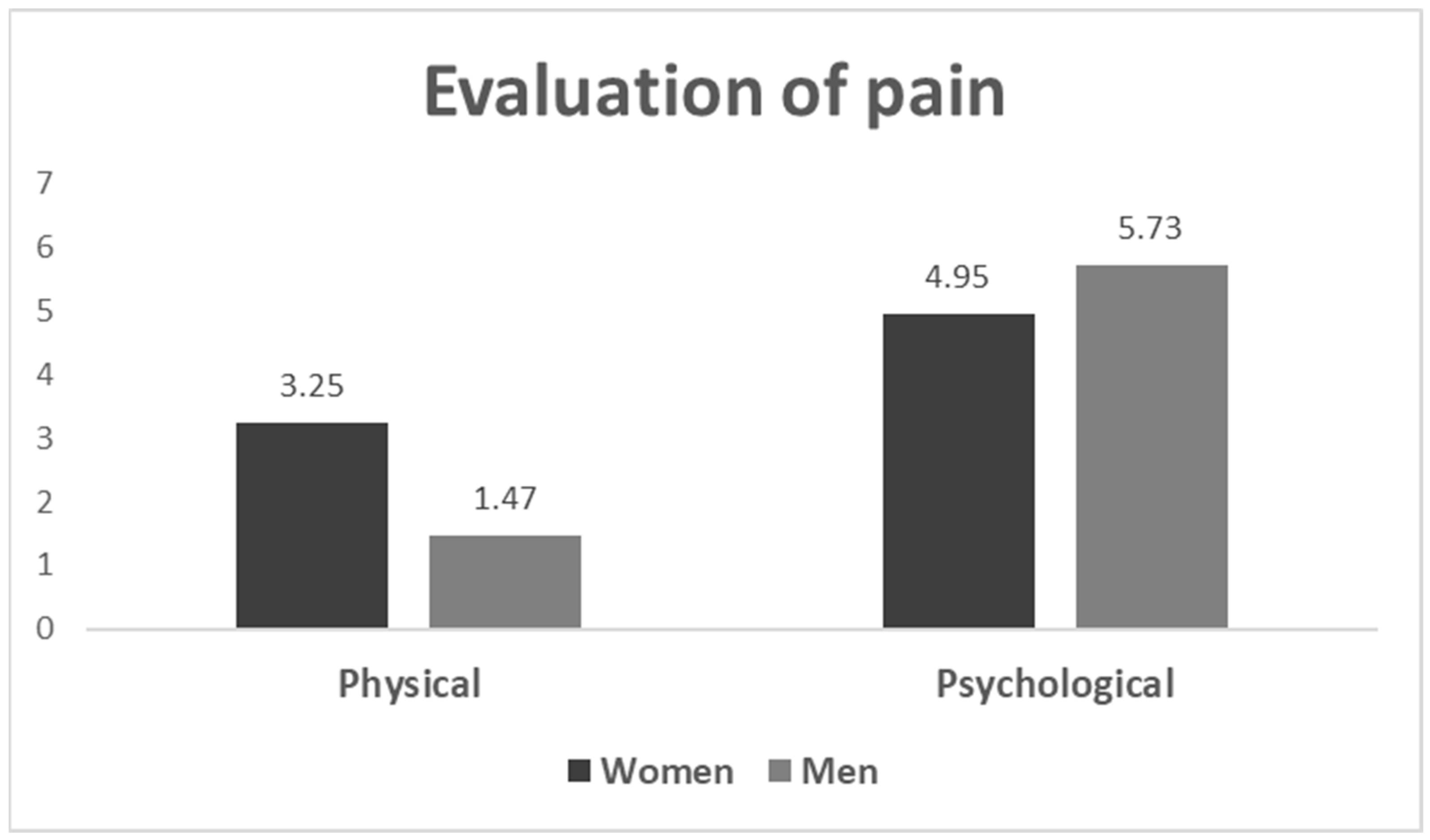The image depicts a black and white bar graph on a white background, titled "Evaluation of Pain." The graph compares men and women in terms of physical and psychological pain. Along the vertical axis, the scale ranges from 0 to 7. On the left side of the graph, it is labeled "Physical," and on the right side, "Psychological."

The bars for women are depicted in a darker color, almost black, while the bars for men are in a lighter gray. For physical pain, the graph indicates that women rate their pain at 3.25, whereas men rate it at 1.47. For psychological pain, women rate their pain at 4.95, and men rate it higher at 5.73. This clearly shows that women perceive physical pain to be more intense than men do, while men perceive psychological pain to be more intense.

The graph is simple yet informative, illustrating the differences in pain tolerance and perception between genders. The specific numerical values offer detailed insights into how men and women evaluate pain differently.